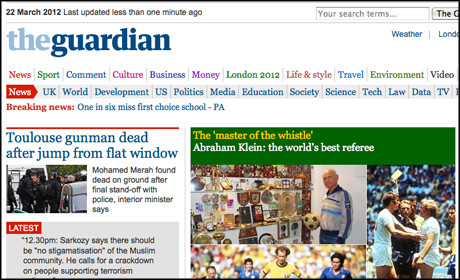A detailed caption for the image:

On March 22, 2012, this web page screenshot from The Guardian showcases a recent update, noted to have been refreshed less than a minute ago. The web page, set against a white background, features The Guardian's logo in the upper left corner, with the "V" in a lighter blue and "Guardian" in a darker blue. Centrally located towards the bottom right, there is a picture box labeled "The Master of the Whistle: Abraham Klein, the World's Best Referee." This box contains four images: a man holding a soccer ball, two soccer players facing a referee with one player placing his hands on the other’s chest, and additional scenes not fully detailed. To the left of this collection, there's an advertisement headlined "Toulouse Gunman Dead After Jump from Flat Window," accompanied by an image likely showing police at the scene, with visible hues of green, red, and blue interspersed throughout the page, contributing to the vibrant visual palette.